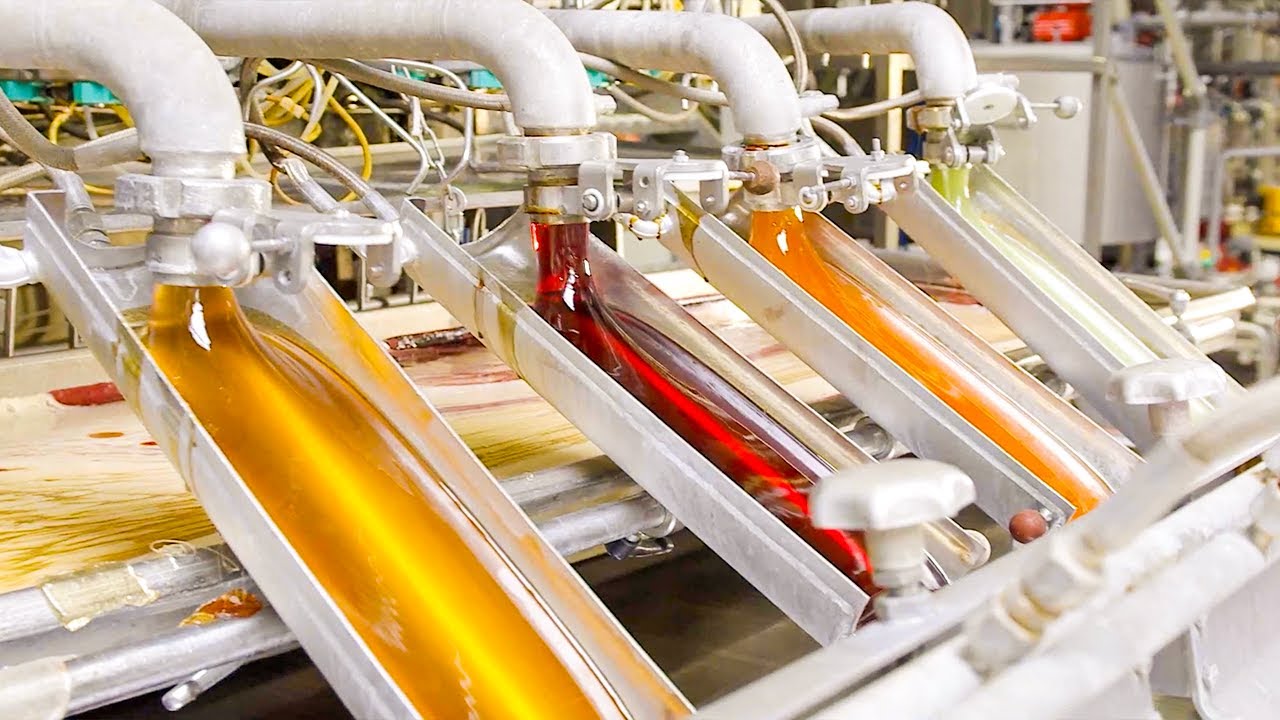The image shows a real-life factory setting where four white hoses curve downwards, dispensing brightly colored, thick, and viscous fluids onto an angled metal conveyor belt. The fluids are distinctly different in color: the hose furthest to the left releases an orange-yellow liquid, the next to the right dispenses a dark burgundy fluid, followed by an orange liquid, and the furthest to the right emits a slightly green fluid. The background is filled with various factory apparatuses, including gray and white pipes and tubes, and there are multiple containers, canisters, and a large conveyor belt that appears to carry items resembling sticks or pasta. The scene is zoomed in, focused on the machinery with no humans present, highlighting the intricate wiring and industrial components involved in the production process.